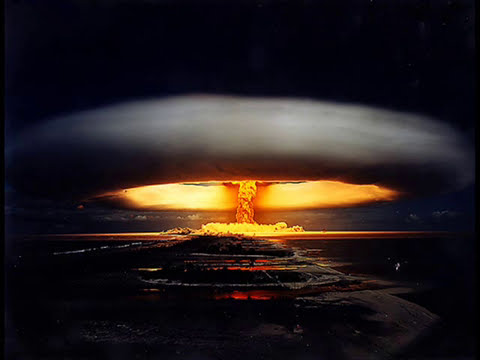This photograph captures the catastrophic moment of a nuclear explosion, depicted in vivid detail. The scene is set at night, with the bottom third of the image showcasing a dark, expansive body of water, possibly with mountains or an island in the distance. The city spans across the image, viewed from an elevated perspective. At the center of the image, the intense initial blast creates a massive, fiery mushroom cloud, radiating shades of orange, yellow, and red. This explosion dominates the scene, with its bright light reflecting off the city and the water below. The upper half of the image features a disc-shaped, black and gray cloud, with the inside appearing almost like molten lava due to the vibrant colors. The fiery smoke extends upwards along the halfway point of the image, adding to the dramatic effect. Overall, the explosion is immense, occupying most of the photograph and suggesting a scene either from a graphic rendering or a real event, portraying a powerful moment of destruction.